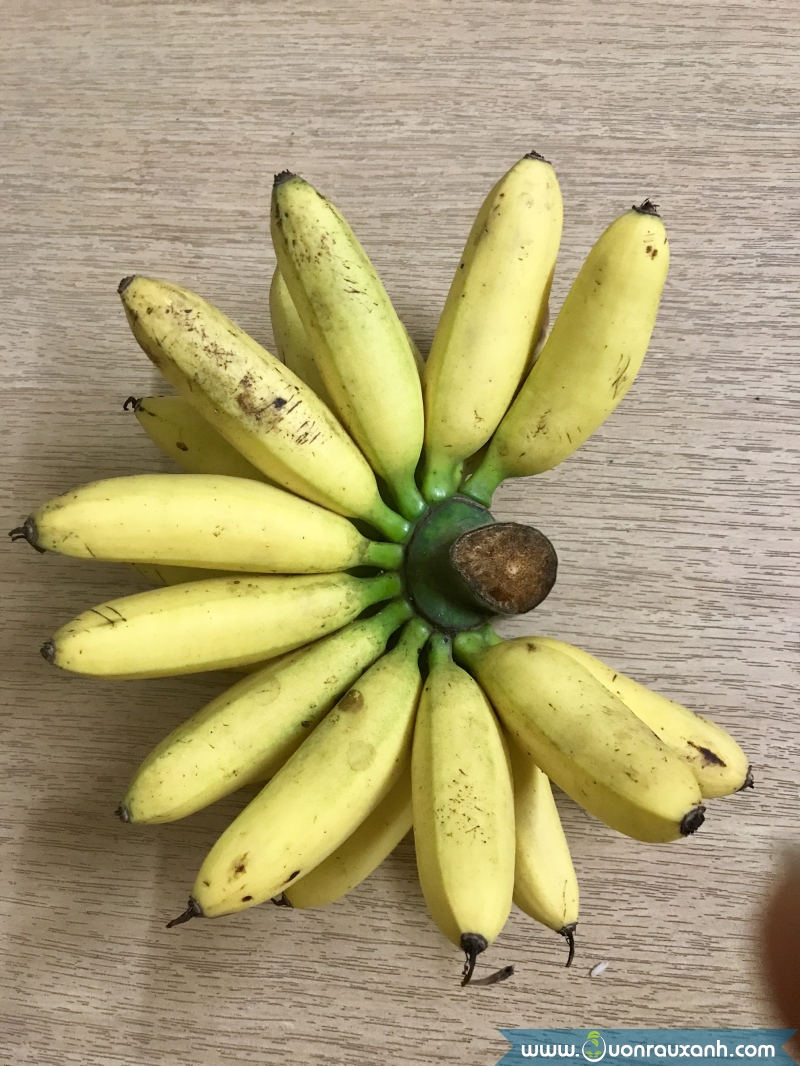The image depicts a top-down view of a kitchen tabletop made of tan-colored wood with small brown and black stripes running across the surface. Centered in the photograph is a spiral arrangement of numerous light yellow ladyfinger bananas. The bananas are primarily light yellow with green stems, some yellow scuff marks, and dark brown tips. The central stem of the banana bunch is dark green with a chocolate brown cut end. Below the bananas, the tabletop appears somewhat artificial with a soft dusty light brown hue and light stippling. At the bottom right of the image, there is a watermark that reads "www.uonrauxanh.com" in white text on a transparent blue ribbon. The overall scene showcases a harmonious collection of at least 15 bananas, likely more, arranged together on the patterned wooden surface.